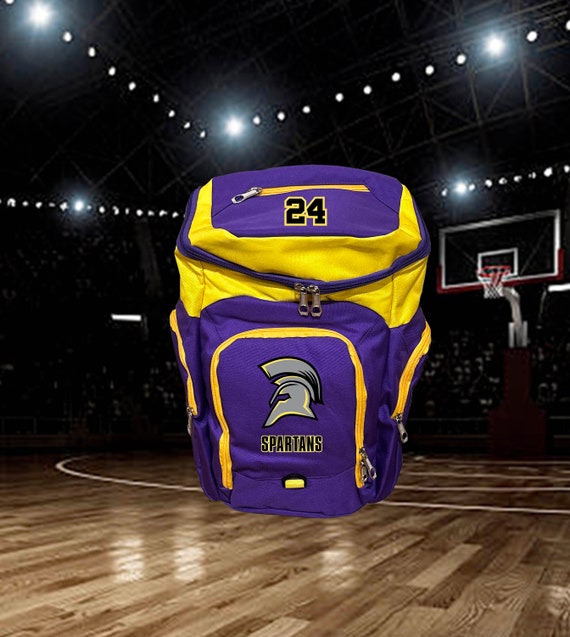This is a product advertisement photograph featuring a purple and yellow backpack, which appears to be a tribute to Kobe Bryant due to the number 24 prominently displayed in black, outlined in yellow, at the top of the bag. The backpack has "Spartans" written on the front pocket, accompanied by a silver helmet logo with yellow trim. The image is set in a dimly lit basketball arena, with the highly polished hardwood floor of the court, white floor markings, and a professional basketball hoop with a glass backboard visible in the background. The arena's rafter lights are faintly visible above, casting small, bright points of light across the scene, while the crowd is suggested but remains shrouded in shadow. The photograph uses a portrait orientation, drawing attention to the detailed design of the backpack and its vibrant colors against the darker, dramatic setting of the court.